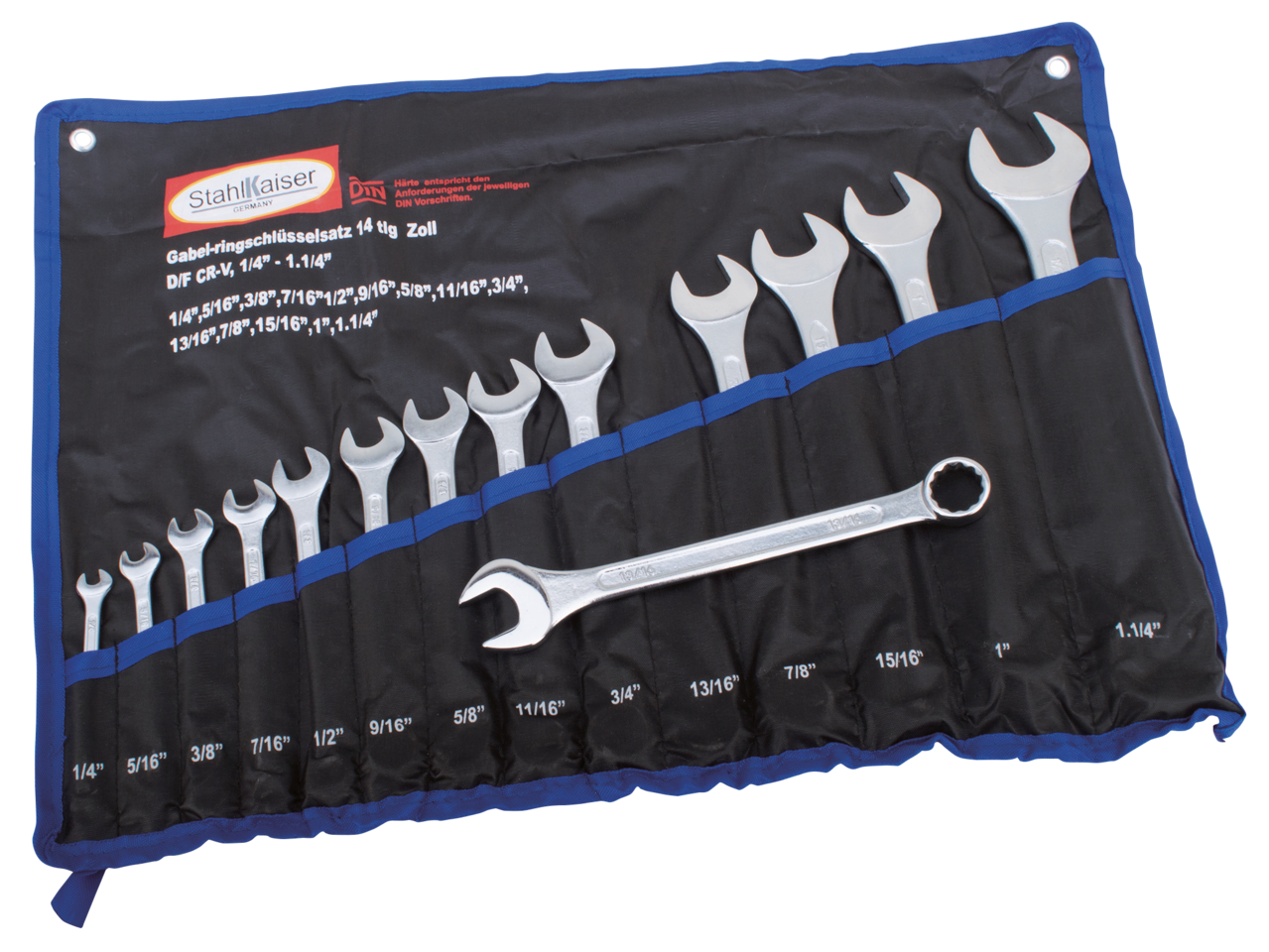This photograph shows a Stahl-Kaiser wrench tool kit, meticulously presented on a white background. The black vinyl pouch, accented with light blue borders, houses a comprehensive set of wrenches ranging from 1/4 inch to 1 1/4 inches in size. Each shiny chrome wrench fits neatly into individual slots, marked with their respective sizes to ensure easy organization. One wrench, the 13/16 inch, is laid on top of the pouch for closer inspection. The Stahl-Kaiser logo is prominently displayed in a white oval contained within a black rectangle, situated on the front of the kit. Below the tool kit, the Zodiac watermark appears in gray lettering inside an oval shape, indicative of an additional layer of branding. This versatile tool kit is designed for portability, capable of being rolled up for transport or storage, making it ideal for mechanics and carpenters alike.